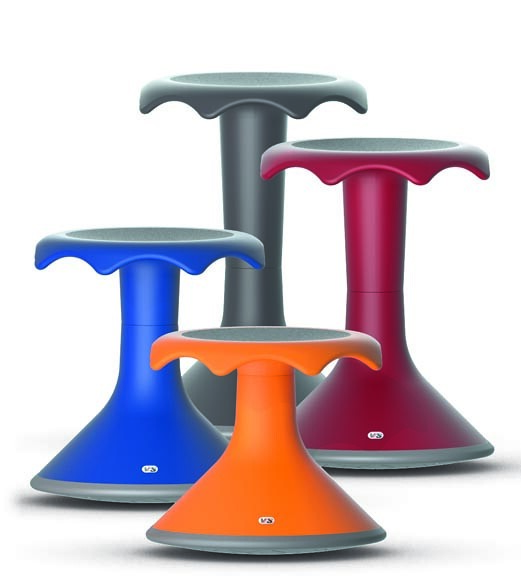The image features four modern stools arranged in varying heights against a plain white background. Each stool shares a similar design, featuring a thin base that flares out at the bottom and leads up to a round seat. The shortest stool, positioned in the foreground, is bright orange with a silver metallic detailing at the base. Behind it to the left is a slightly taller stool in dark blue, also adorned with a silver metallic strip at the base. To the right of the blue stool stands a burgundy-colored stool, moderately taller than the previous two, and featuring a similar silver metallic accent. The tallest stool, located in the background, is black and has a triangular-shaped base leading up to its round seat. All four stools share the same circumference but differ in height and color, creating a visually appealing gradient effect as they recede into the background.